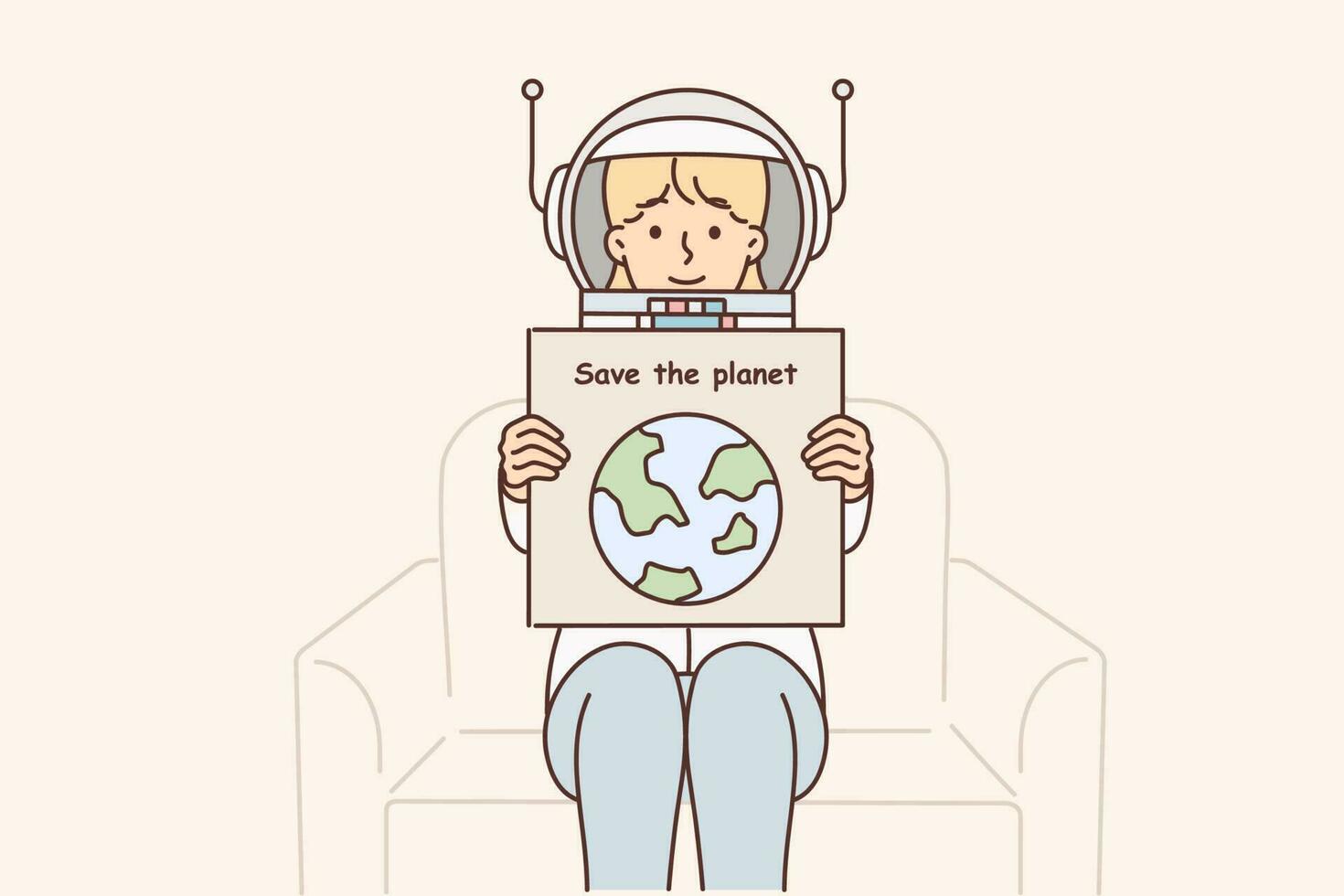This image is a detailed illustration in a simple cartoon style reminiscent of the Herald and the Purple Crayon book, albeit with slightly more detail. The background is a light beige or pinkish color, enhancing the overall minimalistic design. At the center of the image is a young blonde woman, possibly in her teenage years or early twenties, sitting in an outlined armchair with clean, subdued lines. 

She wears an astronaut helmet with two antennae protruding from either side, complementing the futuristic theme. Her helmet features red, blue, and white buttons, and she peers through the rounded glass visor with a smile, emphasizing a friendly and approachable demeanor. The woman is dressed in a white top, possibly a lab coat, and light blue pants, adding muted color contrast to the image.

In her lap, she holds a prominently displayed sign the size of a poster or record album. The sign features a simple, cartoon-like drawing of the Earth, with green landmasses and blue oceans, accompanied by the bold message "Save the Planet." This vivid element stands out, underscoring the environmental message.

Overall, the illustration is vibrant yet clean, focusing on the central figure and her urgent call to action. The minimalist style amplifies the visual impact of the depicted elements, making the plea to "Save the Planet" both clear and compelling.